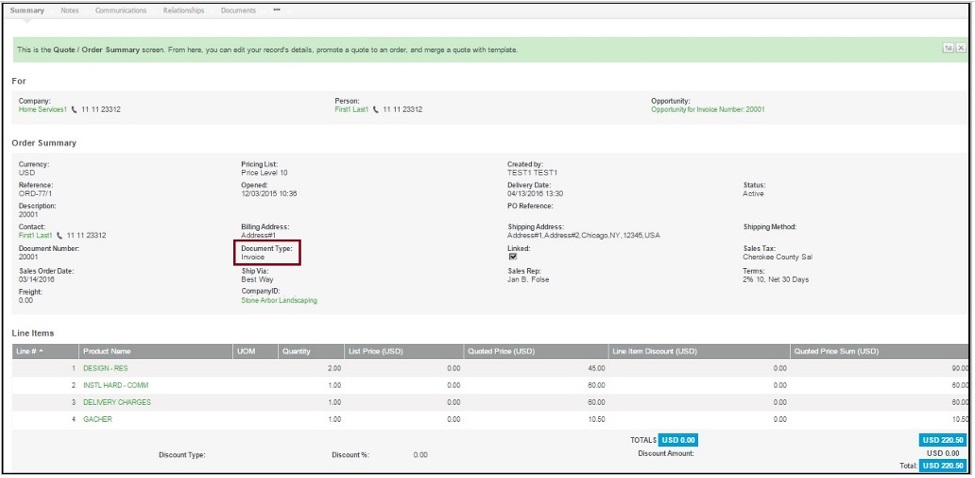This is a detailed order summary screenshot, displaying a cropped view of a quotation interface. At the top, there are navigation categories labeled as "Summary," "Communications," "Relationships," and "Documents." Below these tabs, a prominent green banner indicates that the screen is for a quote order summary, offering functionalities to edit record details, provide a quote, and merge a quote with a template. An 'X' button to close this banner is positioned on the far right side of it.

Further below, the interface is divided into three main sections. On the far left is a category labeled "For," featuring a green or gray banner that specifies the recipient's company name, and directly beneath it, the company's telephone number is displayed. In the center section labeled "Person," the contact name is provided with their telephone number shown to the right. On the far right, the "Opportunity" section includes text in small green font.

Beneath these sections, the "Order Summary" is clearly marked by a large gray box that details the summary information. Notably, a red box highlights the "Document Type" field, indicating that an invoice is the selected document type.

At the bottom of the screen, there is a section for "Line Items," and on the right side, "Total U.S. Dollars" is highlighted in blue. The total amount in U.S. dollars is reiterated at the bottom right corner of the screenshot, highlighted again for emphasis.